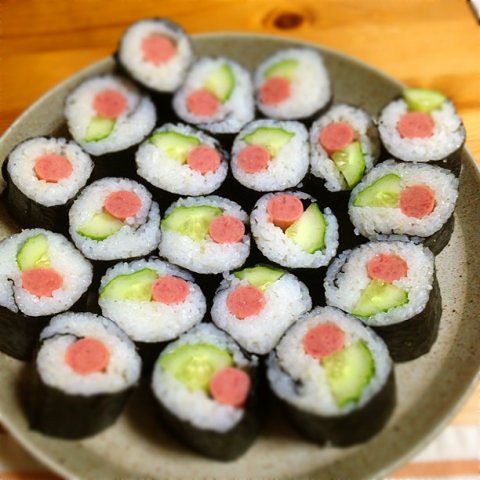This close-up image captures a homemade platter of sushi rolls intricately arranged on a green and gray, speckled circular plate resting on a light brown, wooden table. Each sushi roll features a core of crisp, green cucumber slices paired with a mysterious reddish meat that resembles a beef stick, stacked neatly with pristine white rice and tightly enveloped in dark seaweed. While most rolls include the cucumber, a few only consist of the rice and meat wrapped in seaweed. The bite-sized pieces are sliced restaurant-style and are ready to be served, providing a striking contrast between the detailed textures of the sushi rolls and the natural wood grain of the table beneath them.